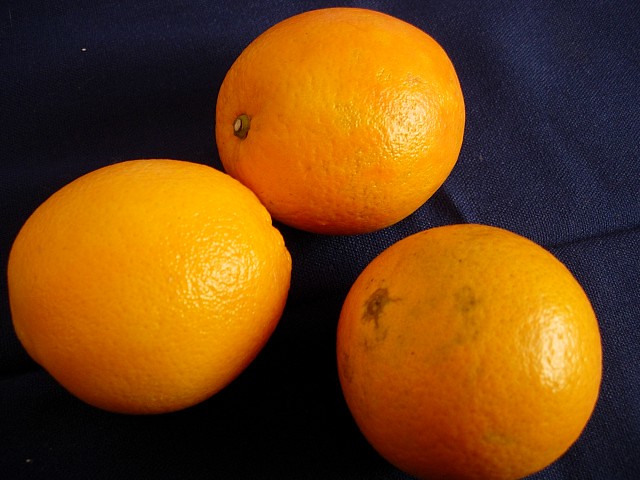This image features a close-up of three oranges arranged in a slightly off-kilter pyramid formation on a navy fabric background. The arrangement forms a triangular pattern with one orange at the top center and two at the bottom. The top orange looks pristine with its stem still attached and no visible blemishes, capturing light on its back-right side. The bottom-left orange shows its flawless skin glistening under the light yet reveals little of its top or bottom. The bottom-right orange exhibits some brownish marks and blemishes. The light, likely coming from the right, emphasizes the texture and color differences among the oranges. A small white speck can be seen on the fabric in the upper-right section of the image.